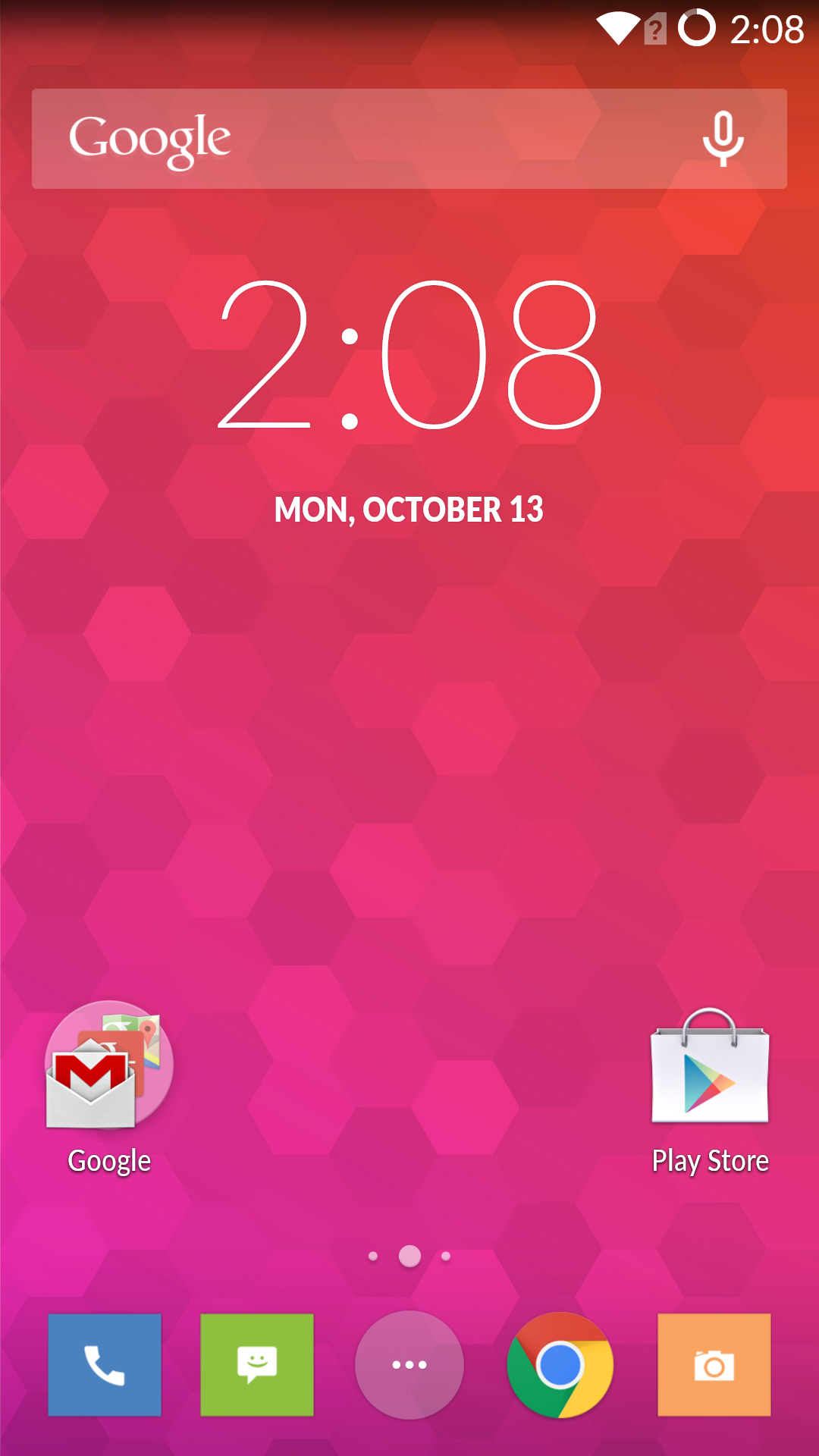The screenshot depicts the home screen of an Android smartphone, likely running either Ice Cream Sandwich or Jelly Bean, as suggested by the distinct fading to black effect on the top title bar. The status bar at the top of the screen provides several indications: the upper left-hand corner is empty, while the upper right-hand corner displays a fully connected Wi-Fi symbol, a grayed-out SIM card icon with a question mark (indicating either no SIM card inserted or an incompatible one), and a custom circular battery indicator showing approximately 90% capacity. Adjacent to these is a clock displaying the time as 2:08, without specifying a.m. or p.m.

Below the status bar, a prominent Google search widget is present, featuring a text box with a microphone icon on the right, allowing users to conduct either typed queries or voice searches straight from the home screen. Centered beneath this widget, the screen prominently shows the current time "2:08" and the date "Monday, October 13th."